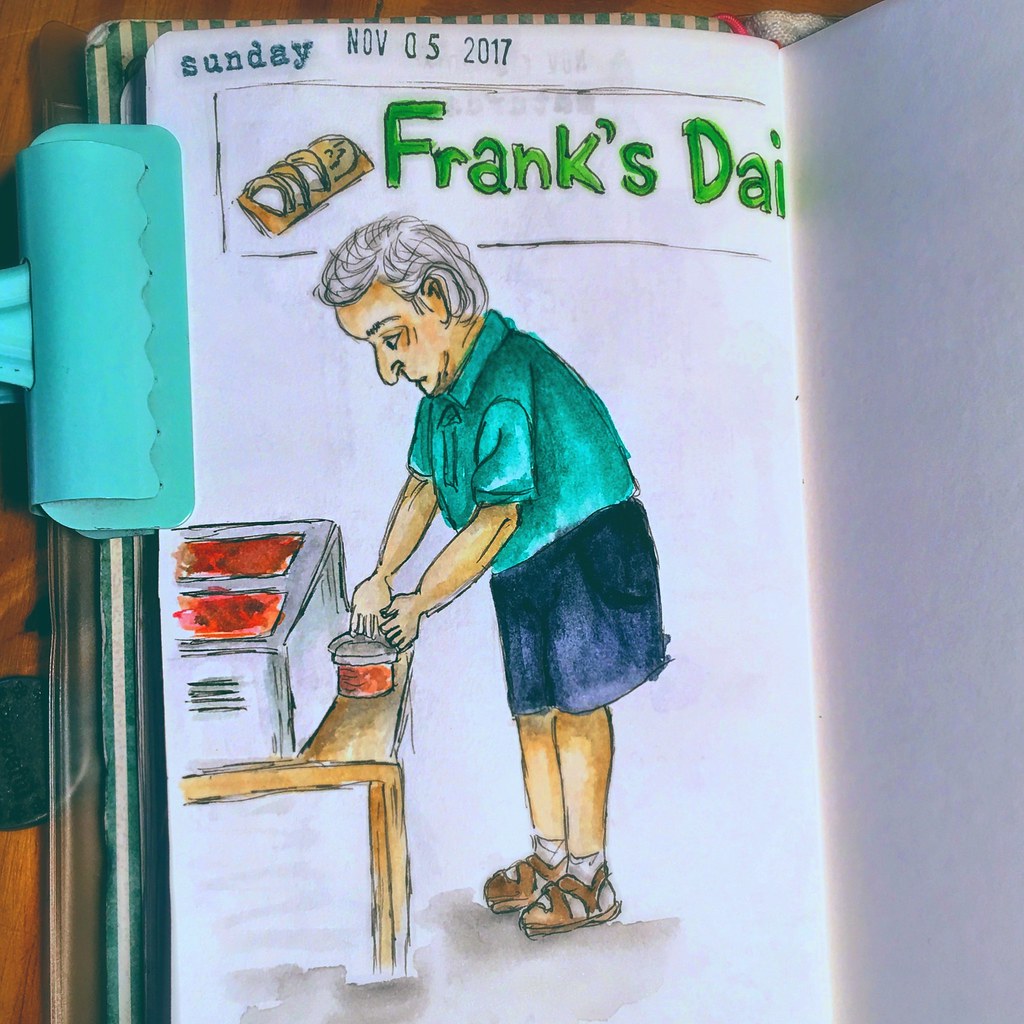The image is a detailed digital drawing or artistic photo resembling a journal entry on plain white, unlined paper, likely created using Procreate or Photoshop. The journal appears to be a teal notebook secured by a turquoise blue clip on the left-hand side. The entry is dated Sunday, November 5th, 2017, and is titled "Frank's D.A.I." in green letters. The centerpiece of the artwork is an older gentleman with white (or gray) hair, donning a turquoise polo shirt and blue (or denim) shorts, along with brown strappy sandals paired with white socks. The gentleman is depicted leaning over what appears to be a low wooden table or countertop, performing a culinary task – possibly putting food into a Tupperware container or trying to open it. In front of him is a silver metal serving dish with two compartments filled with a reddish pinkish food, similar to what he's handling. Accompanying the scene is a small watercolor loaf of sliced bread. The opposite page of the journal is clean and blank.